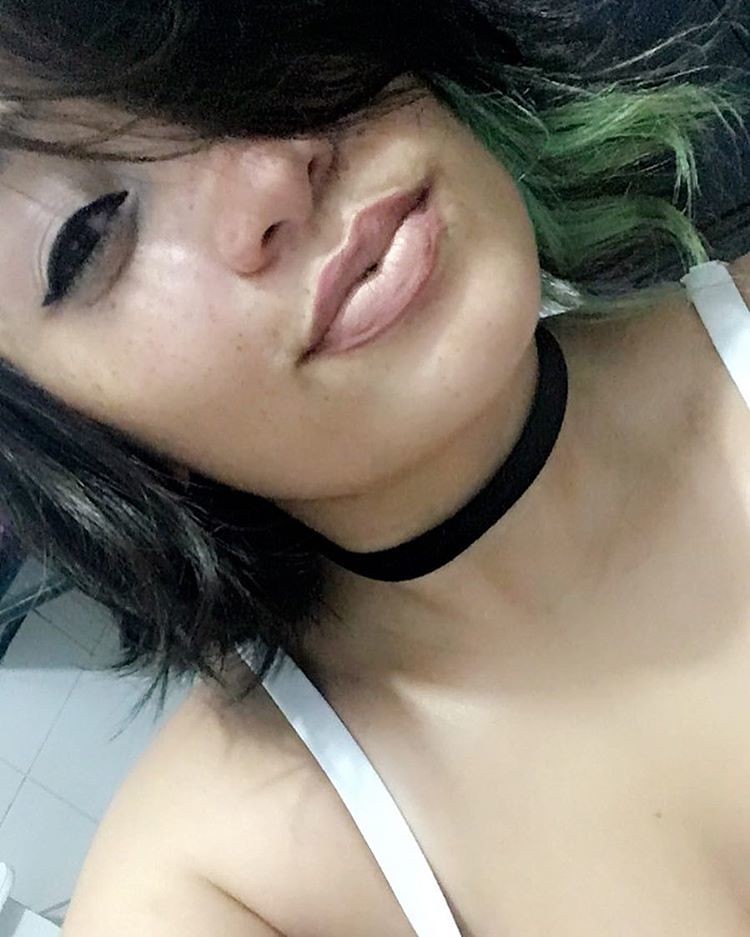The image is a detailed close-up selfie of a light-skinned girl with some freckles, occupying most of the frame. Her face is tilted diagonally, with her head leaning toward the upper left corner and her right shoulder positioned in the lower left. Her black hair, dyed green at the ends on one side, falls over her left eye, partially obscuring it, while her right eye is slightly open as she gazes at the camera with a bemused expression. She has full lips and dark eyes. She is wearing a white halter top, visible by the straps, and a black choker encircles her neck. There is a hint of tiling in the background, though it is mostly out of focus.